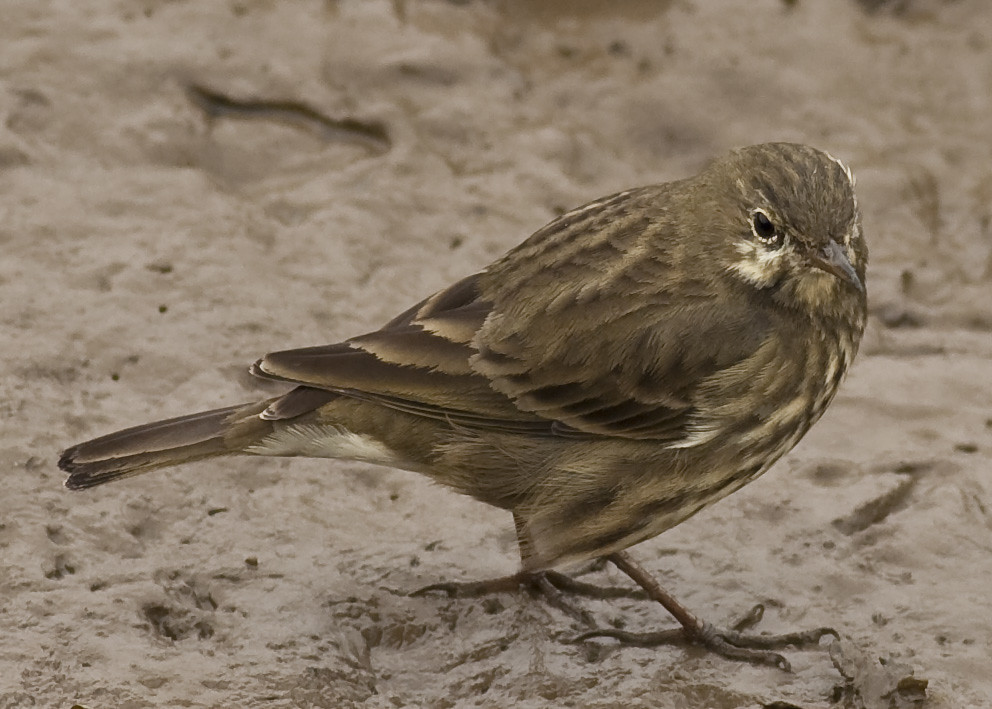The close-up image depicts a small, light brown bird standing on rugged, tan sand. The bird's overall brown plumage is punctuated by significantly darker wingtips and lighter tan, nearly white patches beneath its black eyes. It stands with its wings folded against its back, tilting its head down and to the right, as if inspecting something off-frame. The bird's delicate beak and disproportionately large taloned feet add to its fragile appearance. The sand, recently disturbed or wet, creates a jagged texture underfoot with no other objects or foliage in the background, suggesting an unembellished, natural setting. The bird resembles a tree pipit (Anthus trivialis), recognizable by its coloring and pattern, which aligns closely with illustrations found in ornithological references.